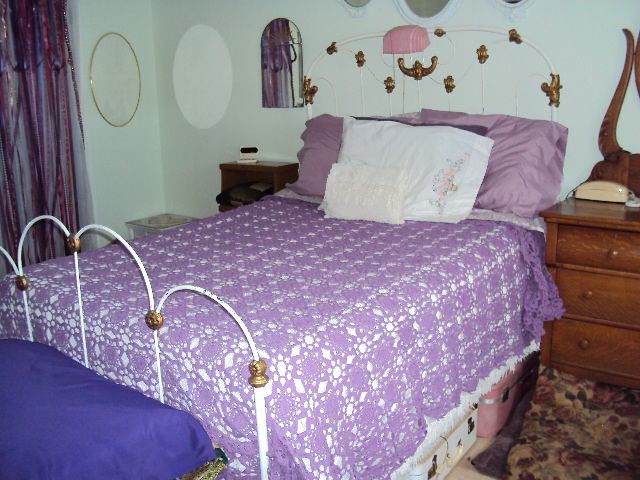The image depicts a vintage bedroom centered around a striking purple bed. The bed features a purple bedspread with a detailed white patterned design of circular grids and diamonds. The bed is adorned with multiple pillows, mostly in shades of purple, including a dark purple or possibly brown pillow partially hidden by white pillows. One of the white pillows has a small, indistinguishable floral print with hints of pink and green. The bed's white wrought iron headboard and footboard boast ornate, flower petal-shaped arcs connected by golden circular elements.

On the left wall, there are two mirrors, one oval and one with an arched top and flat bottom, reflecting light into the room. Above the bed hang three circular items with white frames, likely paintings but partially out of view. A vintage brown wooden dresser with wooden knobs stands to the right of the bed, accompanied by a twisty wooden pattern behind it. A tan, corded landline phone rests on the dresser.

Under the bed are a white suitcase and a pink suitcase. The room features teal walls and an old-looking brown rug with a floral print covering the floor. In the lower left, a blue or possibly indigo pillow is visible. The upper left corner reveals either a curtain or some hanging clothing, adding to the room's cozy, vintage aesthetic.